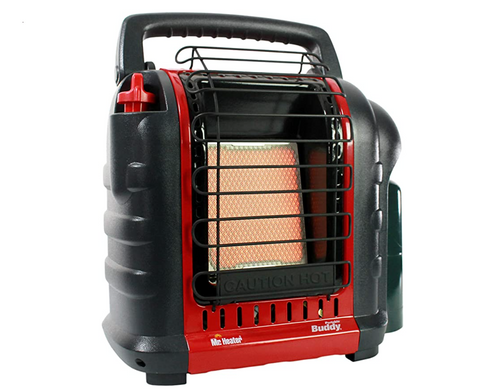This is a detailed photograph of a portable space heater, featuring an industrial and robust design. The heater is encased in a black heavy plastic housing with striking red accents running along its structure. The front of the heater is protected by a black metal grate, which covers the internal heating element—a metallic grid that glows red when in use. This protective grill extends slightly above the heater, ensuring safety by preventing accidental contact with the hot surface. At the top of the heater, there's a black handle for easy portability. The heater's middle section prominently displays the word "Buddy," indicating its brand. Its dimensions suggest it is quite substantial, roughly 3 feet tall, 3 feet wide, and about 6 inches deep. The overall design and features imply it's a high-powered device, possibly battery-operated, suitable for heating spaces efficiently and safely.